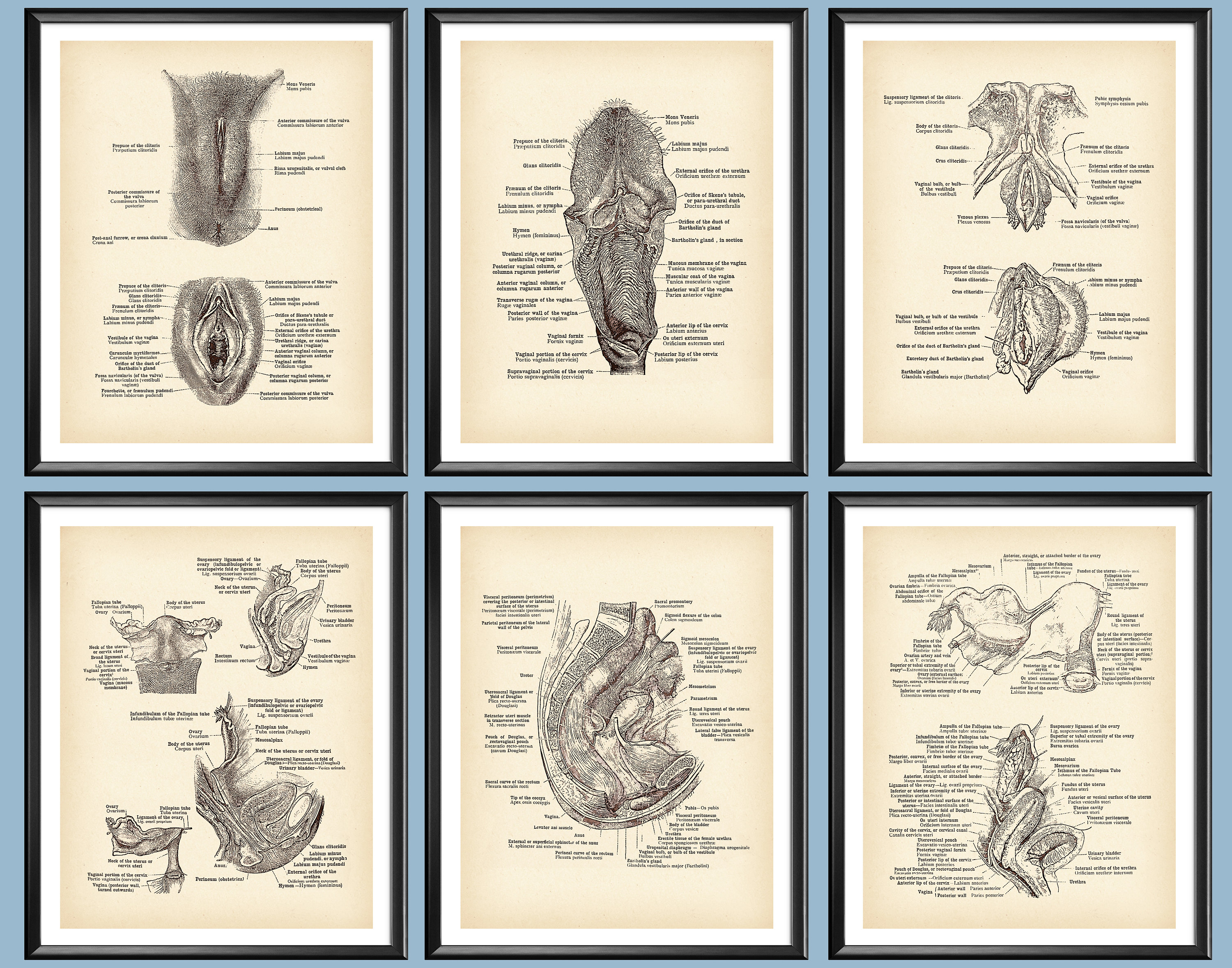This is a composite image of six framed anatomical illustrations displayed against a blue wall. The image, captured in landscape orientation, features two rows of three frames each. Each frame houses a vertical, beige-colored illustration bordered by a narrow white mat and a black outer frame. The illustrations, executed in extremely detailed black line drawings, depict various views of human reproductive anatomy with blowout labels, though the small print is illegible.

In the top left frame, two views of a vulva are shown: the upper illustration displays the labia majora closed, while the lower one reveals the internal structures by pulling the labia apart. The top middle frame likely advances closer to the internal anatomy, possibly featuring parts of the vagina and uterus. The top right frame and the central bottom frame each contain one detailed anatomical view, further expounding on internal reproductive organs.

In the bottom left frame, four illustrations offer various close-up views of different parts of the female reproductive system. The bottom middle frame shows a singular focus, potentially on the uterus itself. The bottom right frame is speculated to illustrate a male penis, among other anatomical features. Each drawing is both scientifically meticulous and artistically rendered, embodying the style of photographic representationalism realism in black and white.